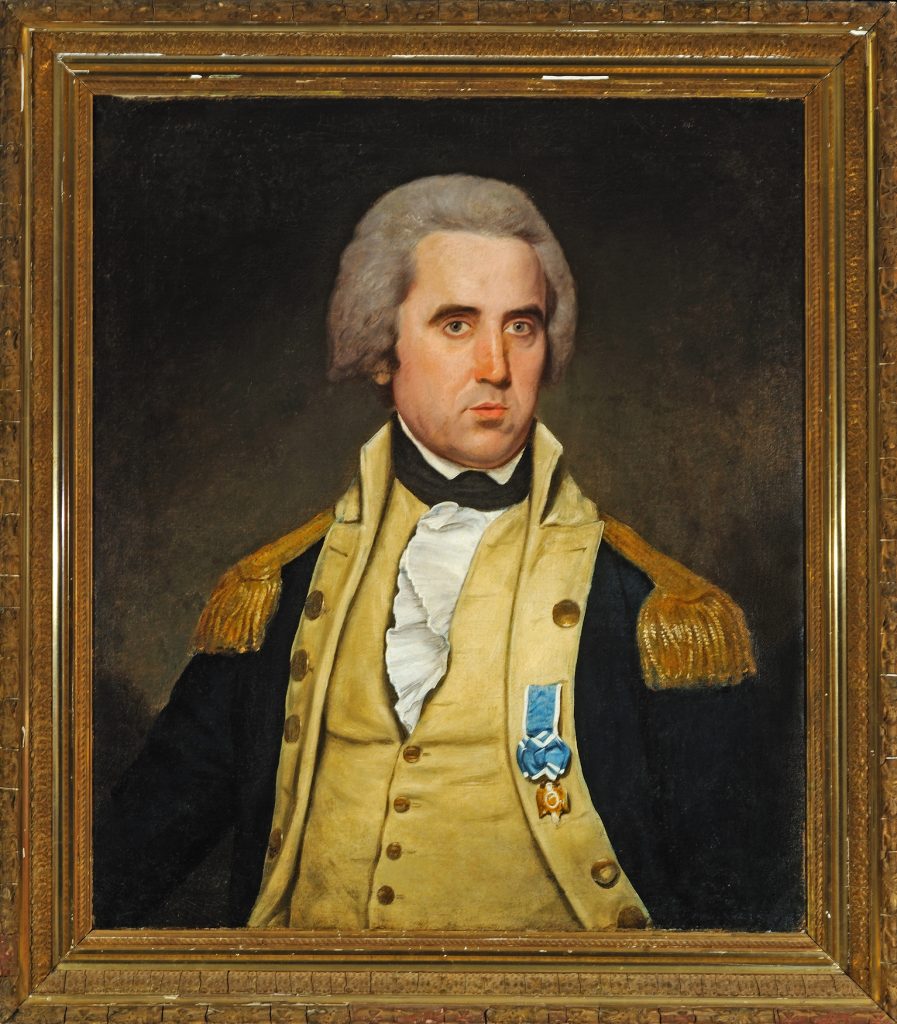This detailed painting portrays a distinguished historical figure, likely a high-ranking general or official from the 1700s to early 1800s, possibly of French origin. The subject is a white man with gray hair and notable features including a long, pointy nose, blue eyes, and dark black eyebrows. He has a small mouth with red lips. His attire is indicative of his high status, featuring a goldish-beige vest adorned with gold buttons, over which he wears a black jacket. The jacket is embellished with gold braids on the shoulder pads and a badge hanging from the collar, hinting at his military or governmental significance. He also wears a shirt with a white ruffled collar and a black tie around his neck. The medals on his chest are blue and gold, adding to the impression of his importance. Behind him is a stark, dark background, and the entire portrait is set within a goldish-bronze frame. His pose shows him facing slightly to the right with his head tilted to the right, while his body tilts slightly to the left, giving a nuanced and thoughtful expression. The painting is a fine example of an oil portrait from its time period.